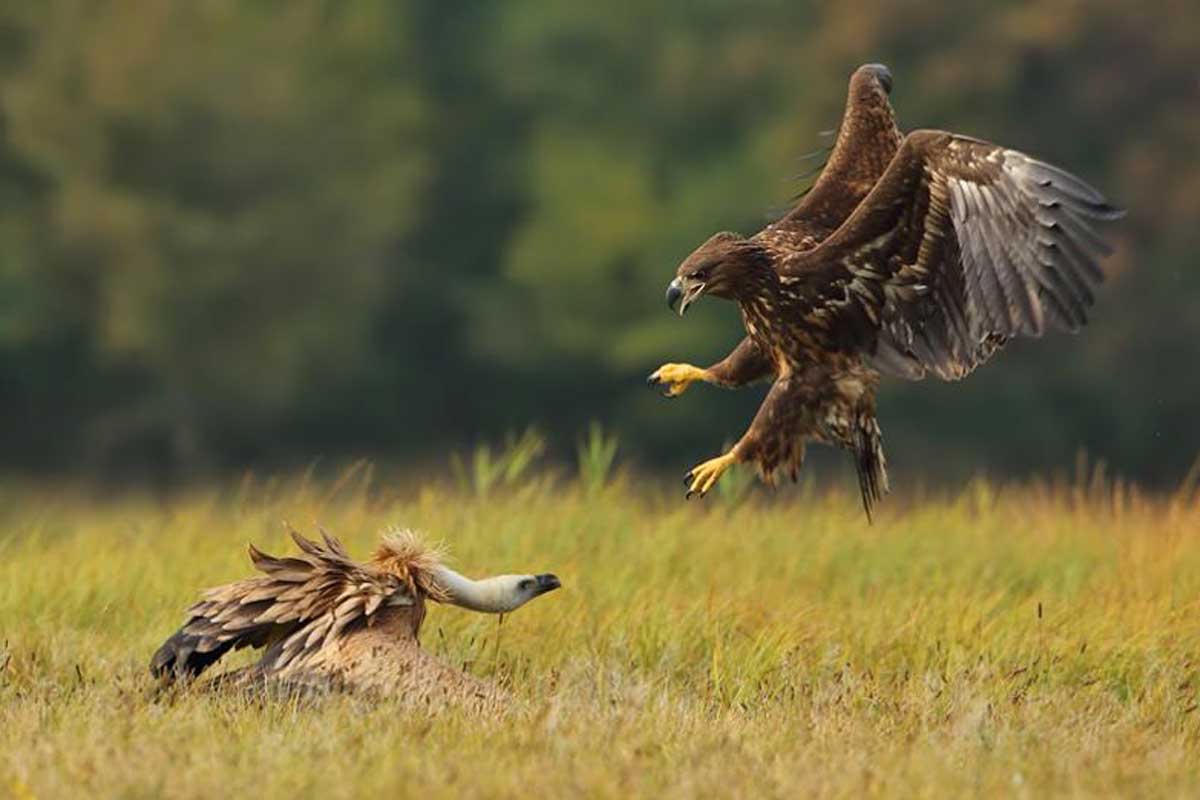In this vivid color photo, the intense action of a predatory encounter is captured in fine detail. It features a dramatic close-up of two birds outside, set against a blurred backdrop of green and brown grass with hints of out-of-focus trees. The primary focus is on the right, where a large, brown hawk with speckled patterns and gray-tipped wings is caught in a rapid descent. Its wings are outstretched and bent, as it prepares to stop mid-air. The hawk's sharp yellow feet are adorned with black talons, ready to strike. Its large, pointed black beak is slightly open, and its fierce gaze is locked onto its target—a bird lying upside down in the grass on the left. This second bird, possibly a buzzard or a duck, is characterized by its ruffled feathers, long neck, and a mix of brown and off-white plumage. With its wings splayed haphazardly and its neck bent, the bird appears lifeless or near death. The hawk, about a foot off the ground and a foot away from its prey, is on the verge of seizing its victim in a display of raw predatory skill.